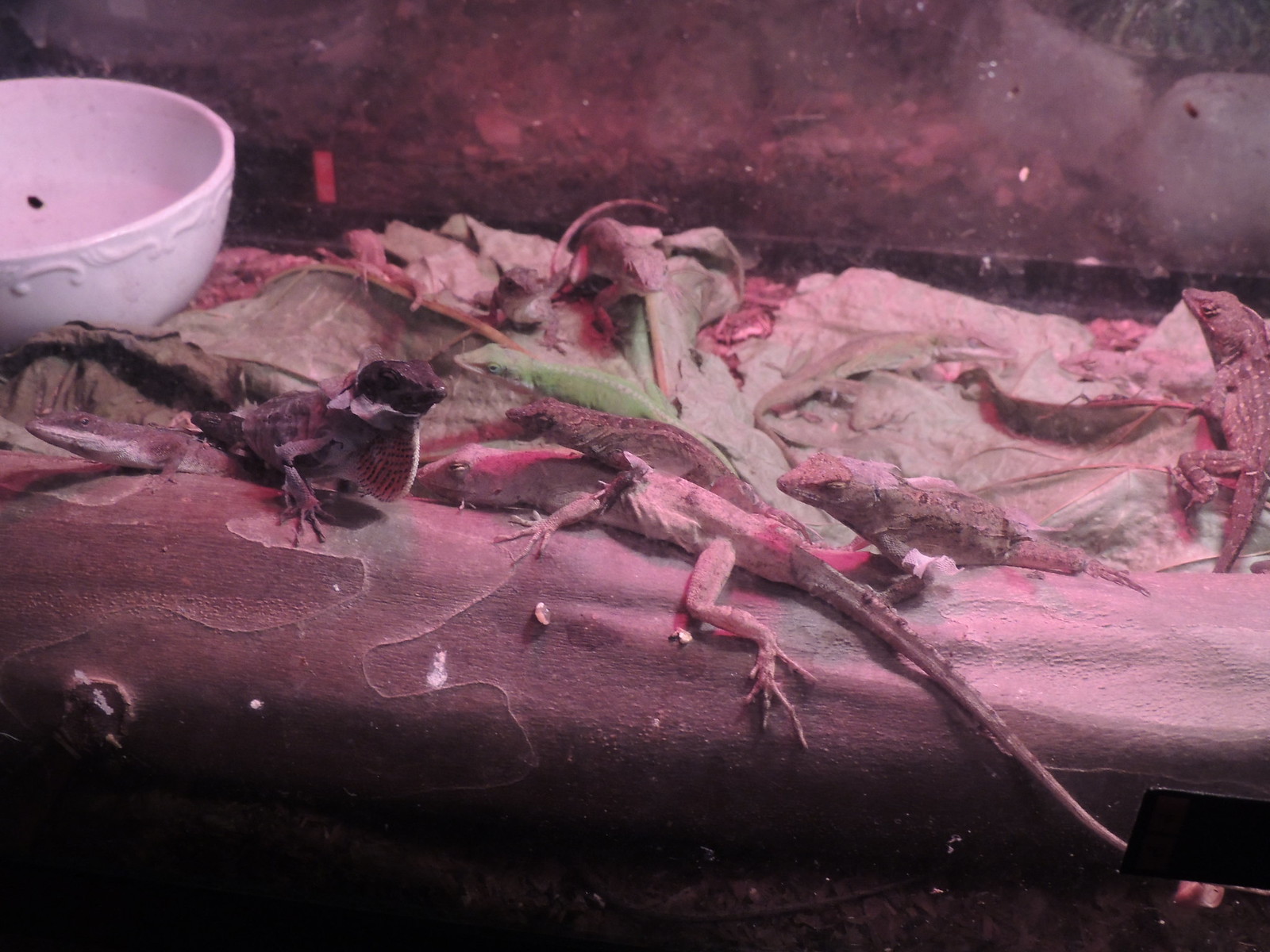The photograph captures the interior of a glass aquarium enclosure housing multiple lizards. The habitat features a wood-like floor with a dark, smoky pink and black hue, possibly illuminated by purple lighting, giving the entire space a reddish-purplish tint. The terrain appears uneven, with rocky formations and a ledge that could be concrete. Numerous lizards of various sizes—small, medium, and large—are scattered across the enclosure. Most of the lizards exhibit colors ranging from brownish to black and tan, with some displaying spots and distinctive designs. Their long, skinny tails and limbs add to their lizard-like appearance, and some of them are in the process of shedding their skin. 

A prominent feature is a log-like decor where a number of lizards are perched. There is also a large white bowl, likely containing water, located in the top left of the frame, adorned with carved, swirly designs along its rim. A mysterious black circle floats within the bowl. In the background, leafy green areas provide additional climbing surfaces for the lizards, and a glass wall reflects the enclosure's interior. Amid the lizards, a small bird with a dark head and a pinkish front can be seen sitting on the ledge, adding to the complexity of this vibrant and lively ecosystem.